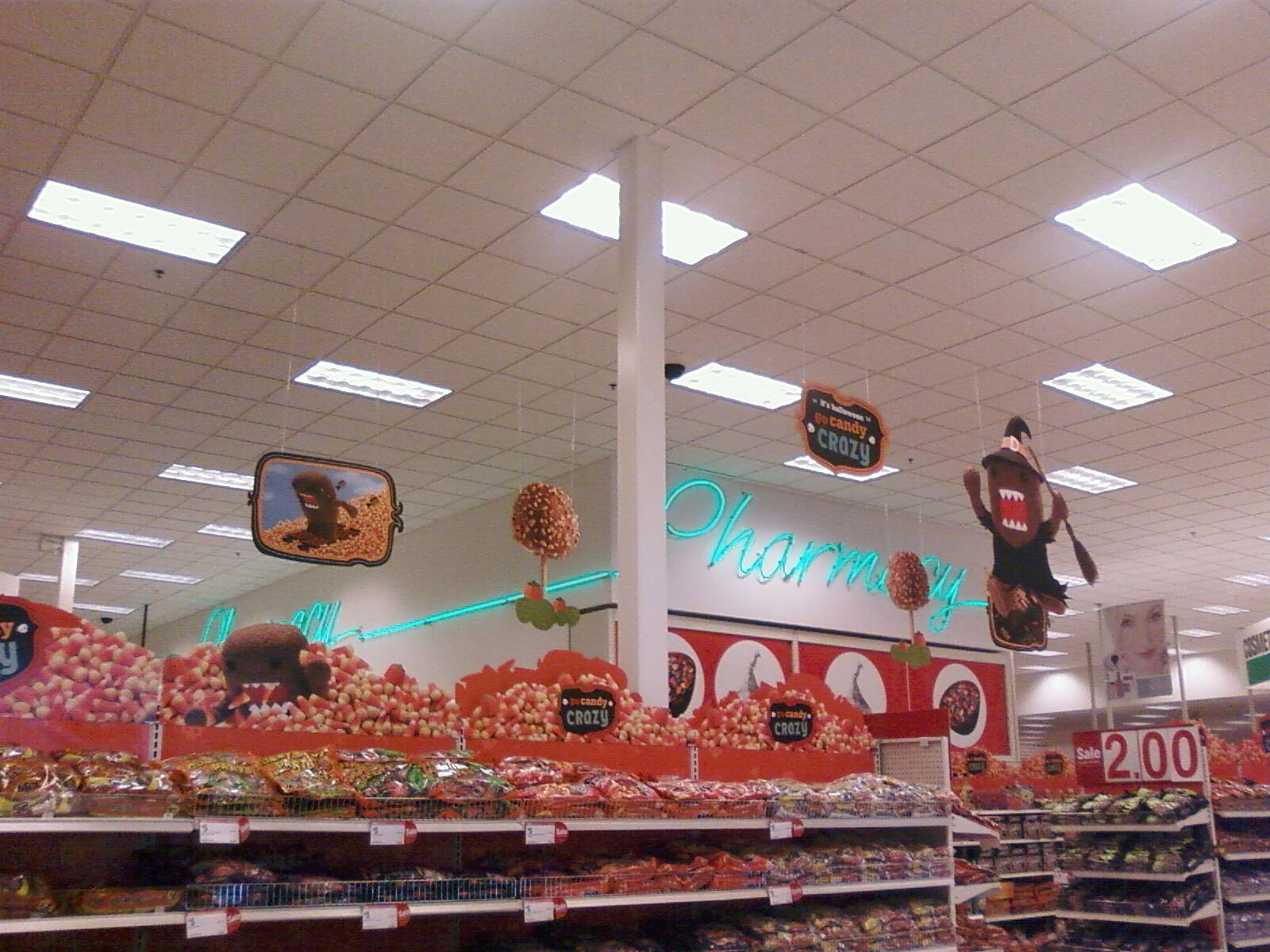The image depicts the interior of a retail store, specifically resembling a candy section, possibly within a Target. The vantage point is from a person standing and looking slightly upward toward the ceiling, which is white and has numerous rectangular fluorescent lights. Hanging from the ceiling are two cutouts featuring a brown mascot with a rectangular head, a red mouth with white teeth, and additional features such as a black hat and a broom. This mascot resembles Domo or perhaps a witch character. 

In the background, a sign with the word "Pharmacy" is displayed in neon blue or turquoise letters on a white wall. The foreground is dominated by well-stocked white shelves filled with various candies in plastic bags, showcasing colors like red, orange, and brown. A prominent $2.00 sign in bold red font on a white background is located at the bottom right of the image. Overall, the scene is bustling with vivid details and a variety of candy items.